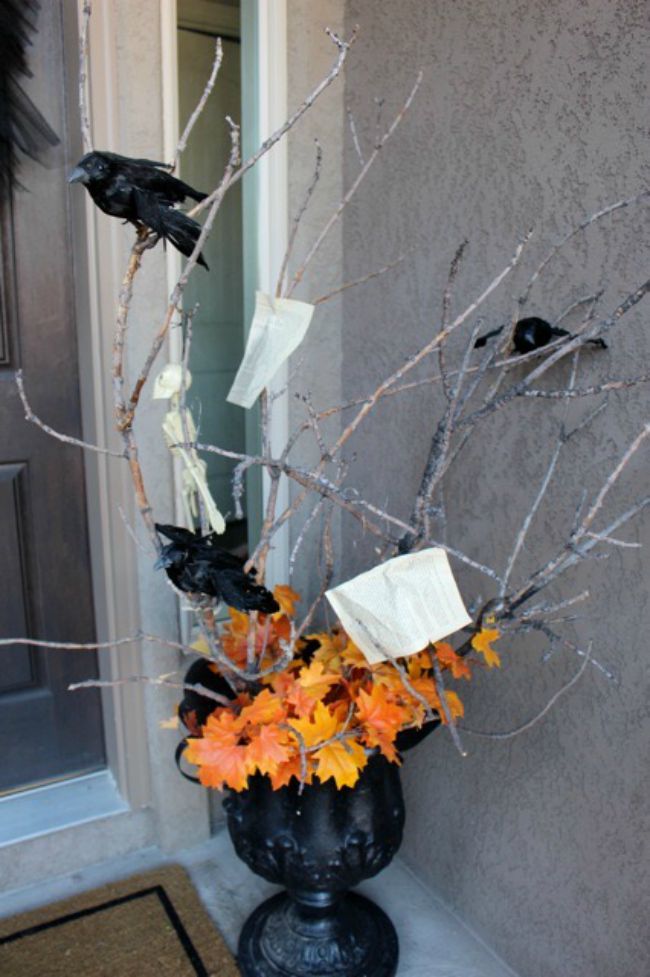This detailed photograph captures the entrance of a house adorned with a striking Halloween decoration. Central to the image is a black door accompanied by a brown, straw-like welcome mat bordered in black. Positioned in the corner where the wall meets the entrance, a black urn sits prominently, evocative of a cauldron. This urn is filled with an arrangement of vibrant orange and yellow fall leaves interspersed with barren branches. Enhancing the spooky aesthetic, the branches are adorned with several white sheets of paper, three realistic-looking blackbirds, and a miniature skeleton figurine. This meticulous composition, from the vivid leaves to the intricate decorations on the branches, conveys a charming yet eerie Halloween vibe.